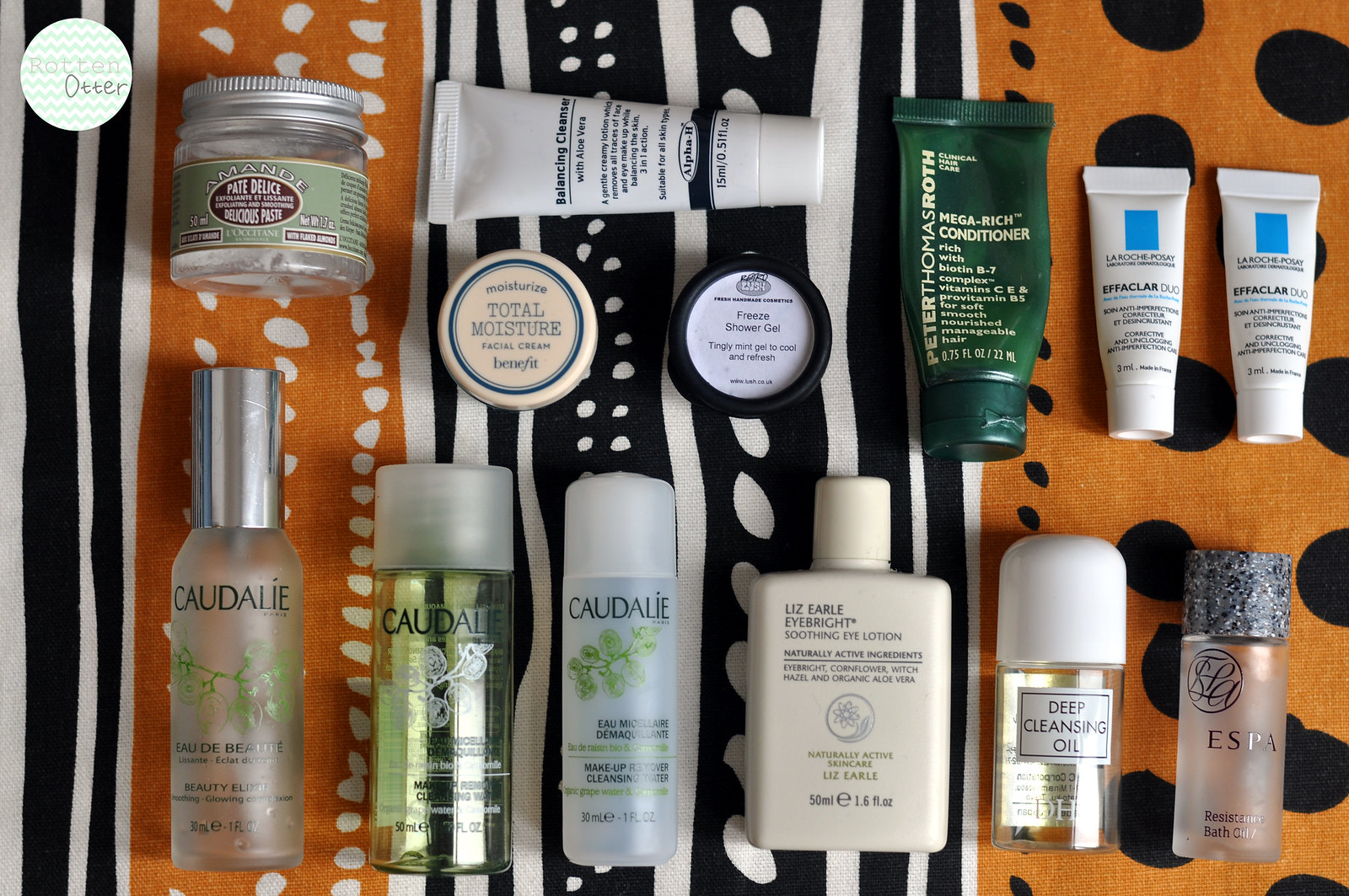This top-down photograph showcases a meticulously arranged skincare collection, artfully displayed on a fabric surface with a vibrant, abstract design. The fabric features an eye-catching mix of orange, black, and white colors, with vertical stripes interspersed with spots of varying sizes, which might be part of a blanket or a piece of furniture.

The skincare products are carefully laid flat and organized into two neat rows, making each item distinctly visible. In the upper-left corner of the image, there's a logo for "Rotten Otter." The logo comprises a circle with a mint green and white chevron pattern background, encasing the words "rotten otter" — "rotten" in a very light gray and "otter" in a darker gray.

The skincare products in the collection include:
1. Benefit Total Moisture Facial Cream
2. Lush Freeze Shower Gel
3. DHC Deep Cleansing Oil
4. A product by Aesop
5. Resistente Bath Oil

The photograph's angle, directly overhead, ensures a clear and comprehensive view of the diverse and curated skincare regimen.